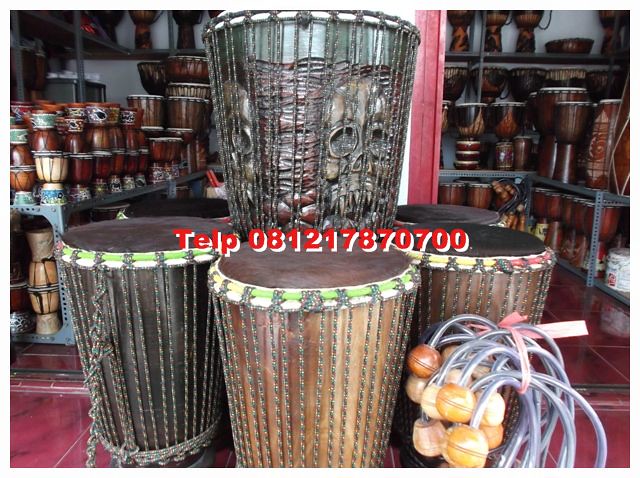The image showcases a vibrant drum shop with an eclectic array of percussion instruments. Dominating the scene is a striking arrangement of four drums in the foreground—three at the bottom, two brown and one black, all encircled by ropes. Atop these sits a blue drum adorned with a skull image. The store's spacious interior features a vast selection of drums, ranging from small to large, all neatly displayed. Highlighted prominently is a red floor that complements the display. Scattered amongst the drums are small maracas or similar musical instruments, adding to the rich musical ambiance. A notable detail is the red text, "TLP 081 21 78 707 00," likely part of an advertisement, subtly integrated into the image. This text suggests contact information, possibly a telephone number, for the shop. The backdrop teems with intricately decorated samba drums, featuring rural art and vivid imagery of dancing figures, enhancing the store's cultural flair.